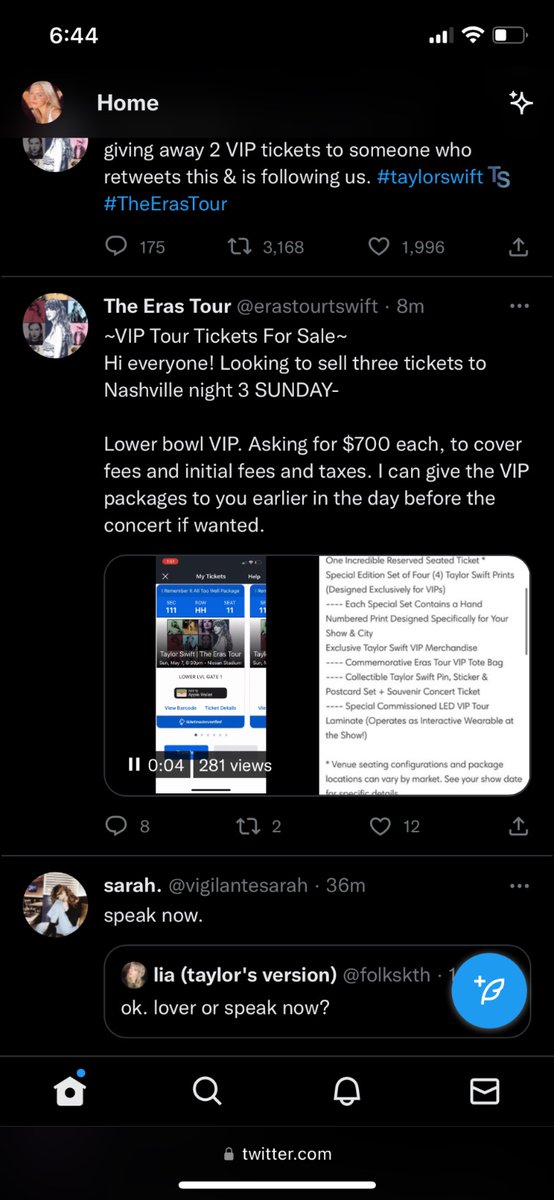The image displays a conversation on a cell phone screen, with a completely black background. At the top, the white text reads "6:44." The battery icon indicates that the battery life is slightly below half, though the exact percentage is not shown. At the top of the screen, it also says "home."

The first visible message includes a partially cut-off profile picture. The message reads: "Giving away two VIP tickets to someone who retweets this and is following us. #TaylorSwiftTS #TheErasTour." 

Below this message, the interaction statistics are visible, showing 176 comments, 3,168 retweets, and 1,996 likes.

The next message reads: "VIP tour tickets for sale. Looking to sell these three tickets to Nashville Night Three (Sunday), lower bowl VIP, asking for $700 each to cover fees and initial taxes. I can give you the VIP packages earlier in the day before the concert if wanted."

At the bottom, there is a video icon followed by a paragraph of text and a message where someone responded with "Speak now," to which another party replied, "Okay, lover or speak now."